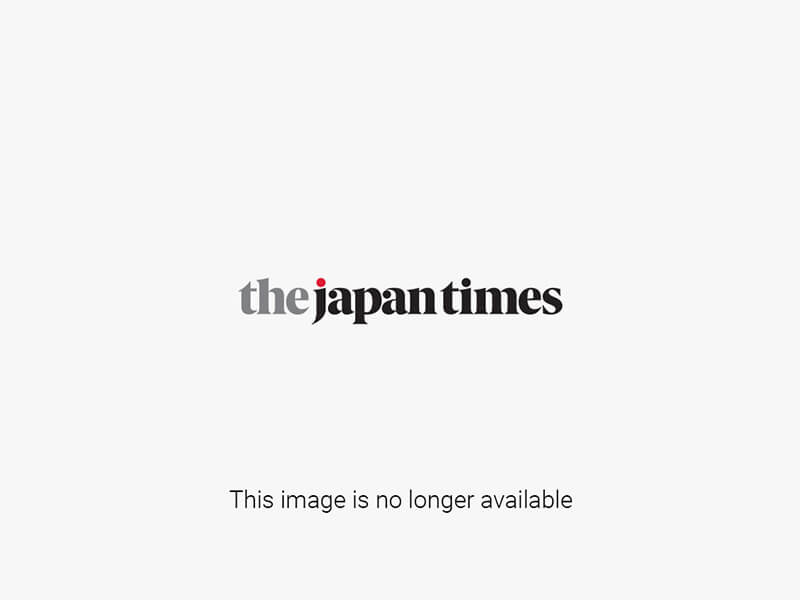This image depicts an outdoor scene featuring a whimsical blue kiosk resembling a small pentagonal cabin or a UFO-themed tourist trap, potentially in Japan, given the Japanese text on a nearby circular blue sign. The sky above is a bright blue with feathery white clouds, and a forested hill forms the backdrop with trees in varying shades of brown and green. 

Foregrounded on the left is the unique blue kiosk with white doors and colorful polka dots in green, blue, white, and red. The kiosk has a distinctive silver saucer-like roof, reminiscent of a flying saucer, and appears somewhat abandoned. A sign, adorned with UFO imagery, a nuclear symbol, and possibly an atom, is attached to a silver and white pole near the kiosk. 

Surrounding the kiosk is a street with light gray sidewalks and a dark gray road featuring two solid yellow lines. The grass in the area appears brownish, with sections of yellow grass around the sidewalk. In the background to the far right, white buildings with black rooftops are visible, further contributing to the quaint roadside scene.